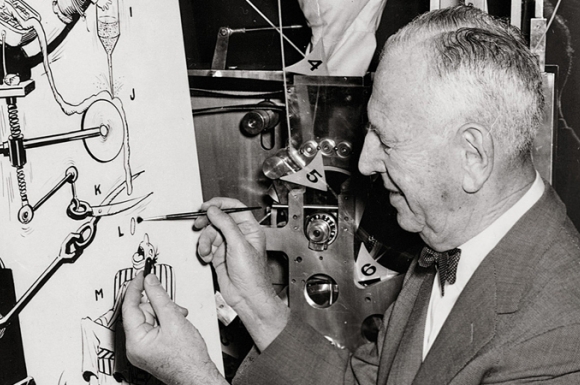This black and white photograph, likely from the 1950s, captures the side profile of an elderly man, probably in his 60s, who is deeply engrossed in illustrating a complex diagram on a large white poster with a paintbrush. The man, who has light skin and gray hair, is dressed in a gray suit coat, a white shirt, and a dark bow tie. He appears to be smiling as he works. The detailed illustration on the poster features a Rube Goldberg-style contraption, including components such as a Rubik's Cube-like device, a pair of scissors cutting a flowing substance, various coils, wheels, and levers, and a man at the bottom in a striped outfit with his mouth open, seemingly ready to consume the liquid or object falling towards him. Behind the elderly man is a machine that mirrors the complexity of his drawing, possibly an old-timey camera or some other intricate device, with numbered arrowheads and a network of strings and levers. The setup suggests he might be recreating or conceptualizing what he sees, perhaps for a cartoon or a scientific illustration.